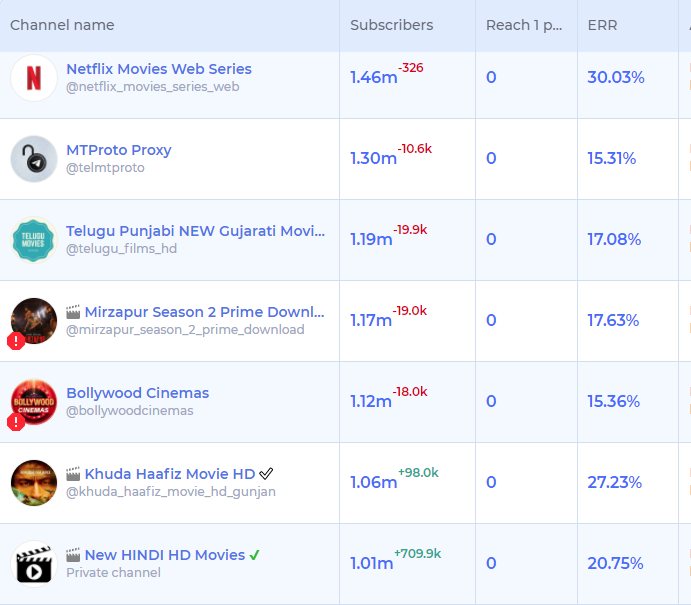A detailed screenshot of a spreadsheet predominantly styled in white and light blue hues. The header row is characterized by a deeper blue shade with grey text, delineating the columns: Channel Name, Subscribers, Reach1P, and ERR percentages.

1. The first entry features the Netflix logo, with "Netflix Movies Web Series" in bold blue text, accompanied by "@NetflixMovies" in smaller grey text below. It records:
   - Subscribers: 1.46M (with a reduction of 326 in red)
   - Reach1P: 0
   - ERR: 30.03%

2. Next is a logo combining a lock and a flying symbol labeled "MTP Rotoproxy" at @MTPProxy. The figures are:
   - Subscribers: 1.30M (with a loss of 10.6K in red)
   - Reach1P: 0
   - ERR: 15.31%

3. Following is a blue-themed logo for "Telugu Punjabi New Gujarati Movie," having the user tag @TeluguPunjabiFilms with:
   - Subscribers: 1.19M (loss of 19.9K in red)
   - Reach1P: 0
   - ERR: 17.08%

4. Another logo with dark colors, depicting a movie icon and a red octagon with a white exclamation mark, is titled "Mirza Per Season 2 Prime Download..." tagged @MirzaSeason2:
   - Subscribers: 1.17M (loss of 19.3K in red)
   - Reach1P: 0
   - ERR: 17.63%

5. The "Bollywood Cinemas" logo, also featuring a red octagon, displays @BollywoodCinema:
   - Subscribers: 1.12M (reduction of 18.0K in red)
   - Reach1P: 0
   - ERR: 15.36%

6. Below this, a logo portrays a person's face with text too small to decipher, along with a movie icon and a white checkmark, titled "Khuda Hafiz Movie HD" @KhudaHafiz:
   - Subscribers: 1.06M (an increase of 98.0K in green)
   - Reach1P: 0
   - ERR: 27.23%

7. The final entry shows a logo with a movie icon and play button, titled "New Hindi HD Movies" with a green checkmark, tagged @HindiHDFilms:
   - Subscribers: 1.01M (a significant gain of 709.9K in green)
   - Reach1P: 0
   - ERR: 20.75%

The spreadsheet meticulously details the performance metrics of each channel, including notable subscriber changes, classified by color coding—red indicating a loss, and green a gain.